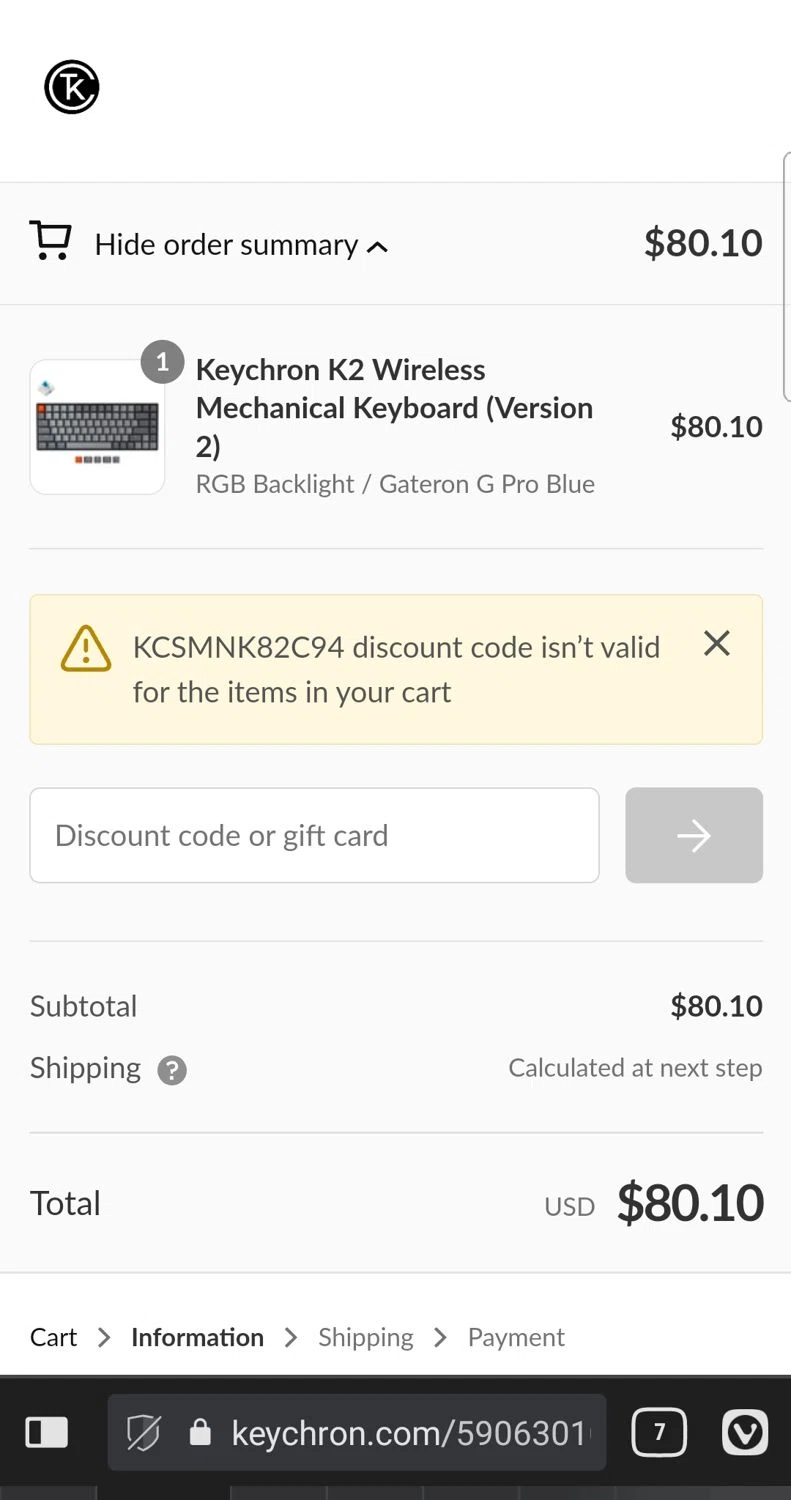This is a cropped screenshot from a mobile phone viewing the Keychron.com website, focusing on the purchasing process for a keyboard. At the top of the screenshot, the Keychron logo is prominently displayed on a white background. Below the logo, there is an expanded "Hide Order Summary" section accompanied by a shopping cart icon. 

Within this section, a thumbnail of the keyboard being purchased is visible on the left side, featuring a grey circle with the number "1" in the top right corner, indicating the quantity. Adjacent to the thumbnail are the product name and details. To the right of these details, the price of $80.10 is clearly shown.

In the center of the screenshot, there's a peach-colored pop-up box containing an error icon and a message stating that the discount code isn't valid for the items in the cart. The box has an 'X' in the top right corner for closing this notification. Below the pop-up, there is a text box for entering a discount code or gift card, featuring a grey arrow button on its right side.

At the bottom part of the page, on the left side, the summary shows "Subtotal," "Shipping," and "Total," with their respective details listed on the right side. The subtotal is indicated as $80.10, with shipping to be calculated at the next step, and the total matching the subtotal at $80.10.